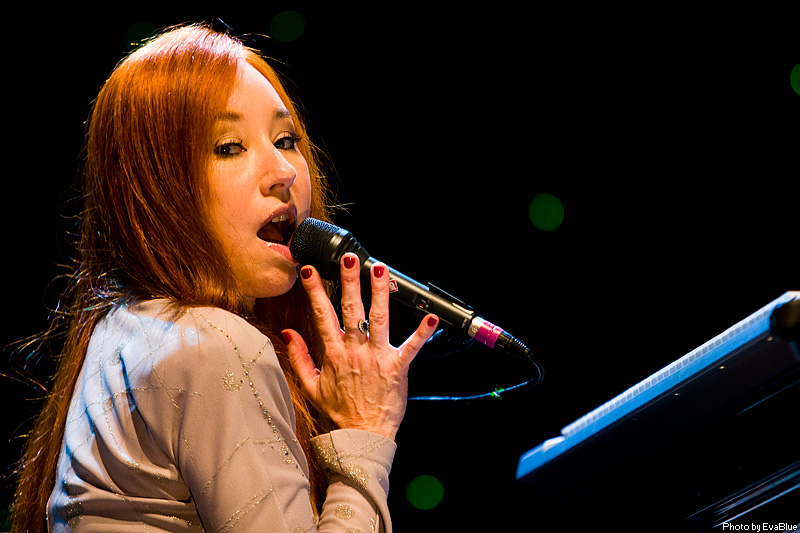The image portrays singer-songwriter Tori Amos in the midst of a performance. She is seated at a black piano, deeply immersed in her music, with her lips close to a black microphone adorned with a red stripe made of paper and a cord trailing from it. Her long, flowing red hair frames her face and falls over her light gray, rhinestone-studded, long-sleeved shirt. Her right hand is on the piano's keyboard while her left hand lightly touches the microphone. She wears a ring with a black gem on her middle finger and her fingernails are painted burgundy. The photograph captures her singing passionately, facing the camera, and looking out into the crowd. The dim, all-black background is accentuated by green light reflections, creating a captivating contrast. There's a small light on the piano, and at the bottom of the image, the credit "Photo by Eva Blue" is visible, indicating the photographer who captured this moment. The setting appears to be a concert, with Tori Amos highlighted under the stage lights.